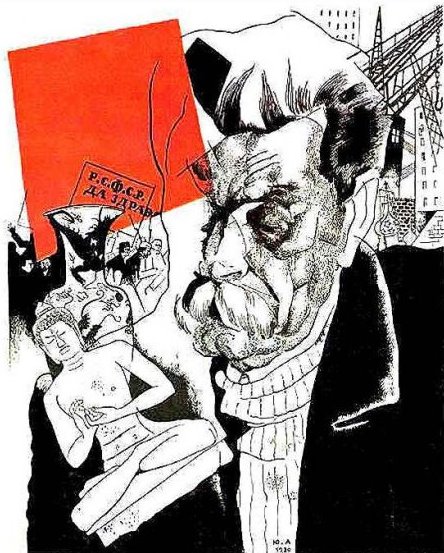The image is a detailed illustration, predominantly black and white with a political cartoon style. At the center is a stern, older man resembling Stalin, characterized by his peppered black and white hair and distinctive mustache with a slight opening in the center. His right eye appears blackened out, and his right cheek is rendered with chalky dots and scales. He is wearing a detailed layered white scarf and a collared black coat that blends into the bottom right and center right edges of the image. The background features a bustling construction site in the top right corner, complete with cranes and buildings, including a white building and a black building with brick walls below them. In the bottom left corner, there is a detailed drawing of a naked Buddha statue with crossed legs and joined hands. Alongside and behind the Buddha, small, indistinct figures and a sign with Russian text can be seen. The top left corner of the image is marked by a large red rectangle, which partially overlaps some foreground elements, adding a striking contrast to the otherwise monochromatic scene.